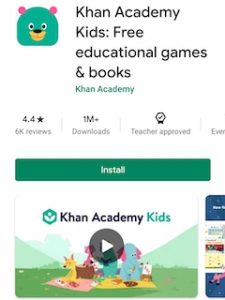This is a detailed screenshot from the Google Play Store, showcasing an educational app designed for children called "Khan Academy Kids: Free Educational Games and Books". The app logo features an animated bear's head in a vibrant turquoise blue color. The bear has two round, pink ears, a yellow snout, and a black nose. Its eyes are large with white sclera and small black pupils.

The title of the app, "Khan Academy Kids - Free Educational Games and Books", is written in black text, with "Khan Academy" repeated below in the same turquoise blue as the bear's head. The app has received 6,000 reviews, earning a rating of 4.4 stars and boasts over 1 million downloads. It is also marked as "Teacher Approved". Users are given the option to install the app or watch a promotional video that provides more information about its features and content.